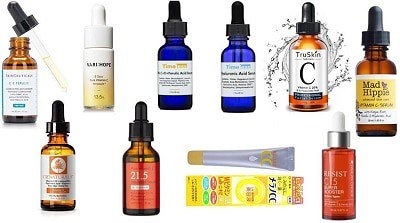This graphic assemblage showcases a diverse collection of facial serums, predominantly centered around the theme of Vitamin C skincare. The array consists of variously shaped and colored tincture bottles and tubes, featuring an assortment of brands and product labels. On the far right, one notable brand, Mad Hippie, makes an appearance, although the text following its name is slightly blurred. Positioned in the lower right corner is the Resist C5 Super Booster, housed in a warm orange-red bottle exuding vibrancy. Adjacent to it is a Japanese lotion tube, opaque in nature, adding an element of intrigue as the liquid inside remains concealed. The tube is displayed outside its box, emphasizing its unique packaging.

Additionally, the collection includes several other tincture bottles, with some crafted from warm brown glass and others from blue glass adorned with white labels. One of the tinctures notably has its dropper removed, showcasing a visible amount of liquid within, adding a dynamic touch to the arrangement. The overall composition is set against a seamless background, emphasizing the variety and sophistication of skincare products, each promising benefits catered to enhancing facial care.